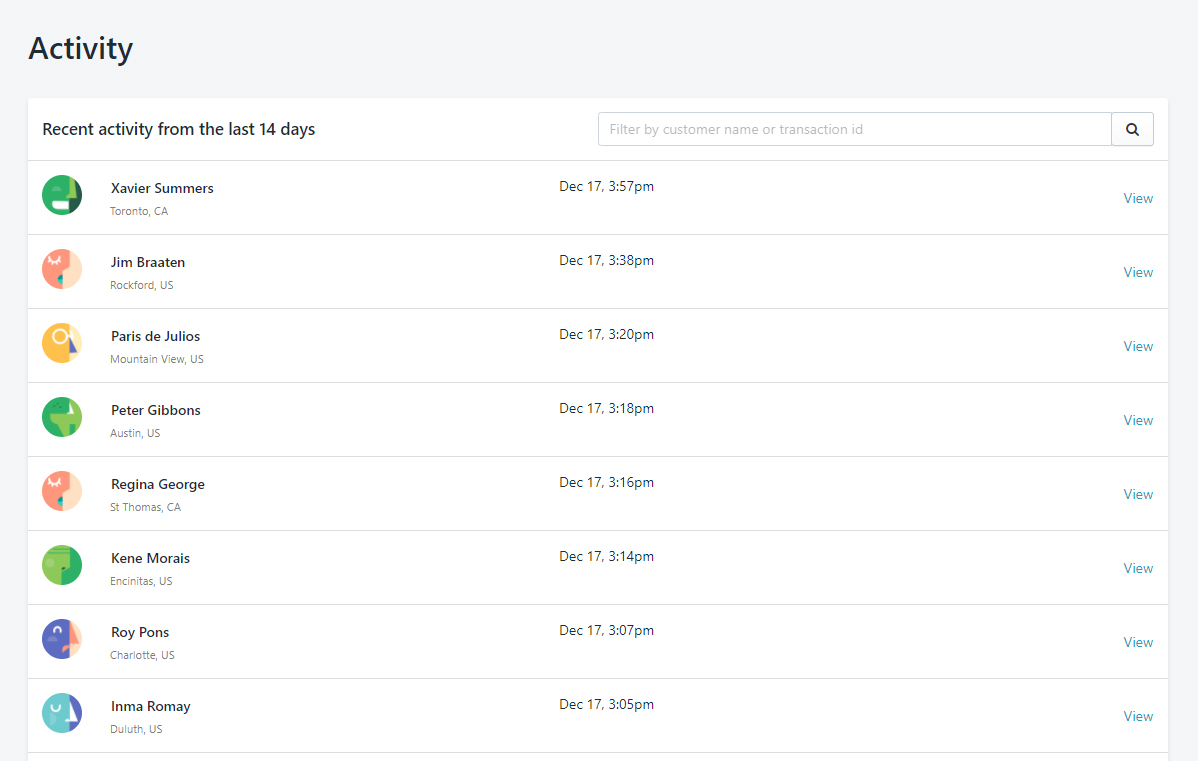The image showcases a screenshot of an activity page, framed by a gray border that is thicker along the top and thinner on the left and right sides. At the top, "Activity" is prominently displayed in bold black text. Directly beneath, within a white box, the text reads "Recent activity from the last 14 days."

On the right-hand side, there is a search bar labeled "Filter by customer name or transaction ID," accompanied by a magnifying glass icon. Below this search bar is a list detailing individual activities, each with a profile icon and specific information.

The activities are listed as follows:

1. Xavier Summers from Toronto, CA, on December 17 at 3:57 p.m. with a "view" option.
2. Jim Brayton from Rockford, US, on December 17 at 3:38 p.m. with a "view" option.
3. Paris T. Julius from Mountain View, US, on December 17 at 3:20 p.m. with a "view" option.
4. Peter Gibbons from Austin, US, on December 17 at 3:18 p.m. with a "view" option.
5. Regina George from St. Thomas, California, on December 17 at 3:16 p.m. with a "view" option.
6. Canamore AS from Sanitas, US, on December 17 at 3:14 p.m. with a "view" option.
7. Roy Pawns from Charlotte, US, on December 17 at 3:07 p.m. with a "view" option.
8. Inn My Rooma from Duluth, US, on December 17 at 3:05 p.m. with a "view" option.